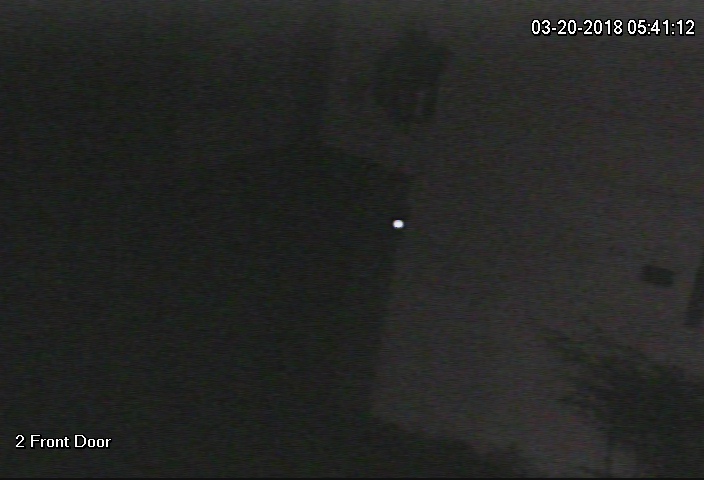The image, seemingly captured by a security camera, is cloaked in near-total darkness, suggesting it was taken at night. Despite the low visibility, the faint outlines of a room are discernible. On the right side, a white wall is faintly visible, appearing to form a recessed area resembling a hallway that converges towards the center of the frame. Near the upper center of the image, you can just make out the outline of a wall and a door. Notably, in the bottom left corner, white text reads "front door," indicating the camera's location. A barely visible white dot can be seen in the middle of the image. In the upper right corner, the timestamp is displayed, showing the date "03-20-2018" and the time "05:41:12."